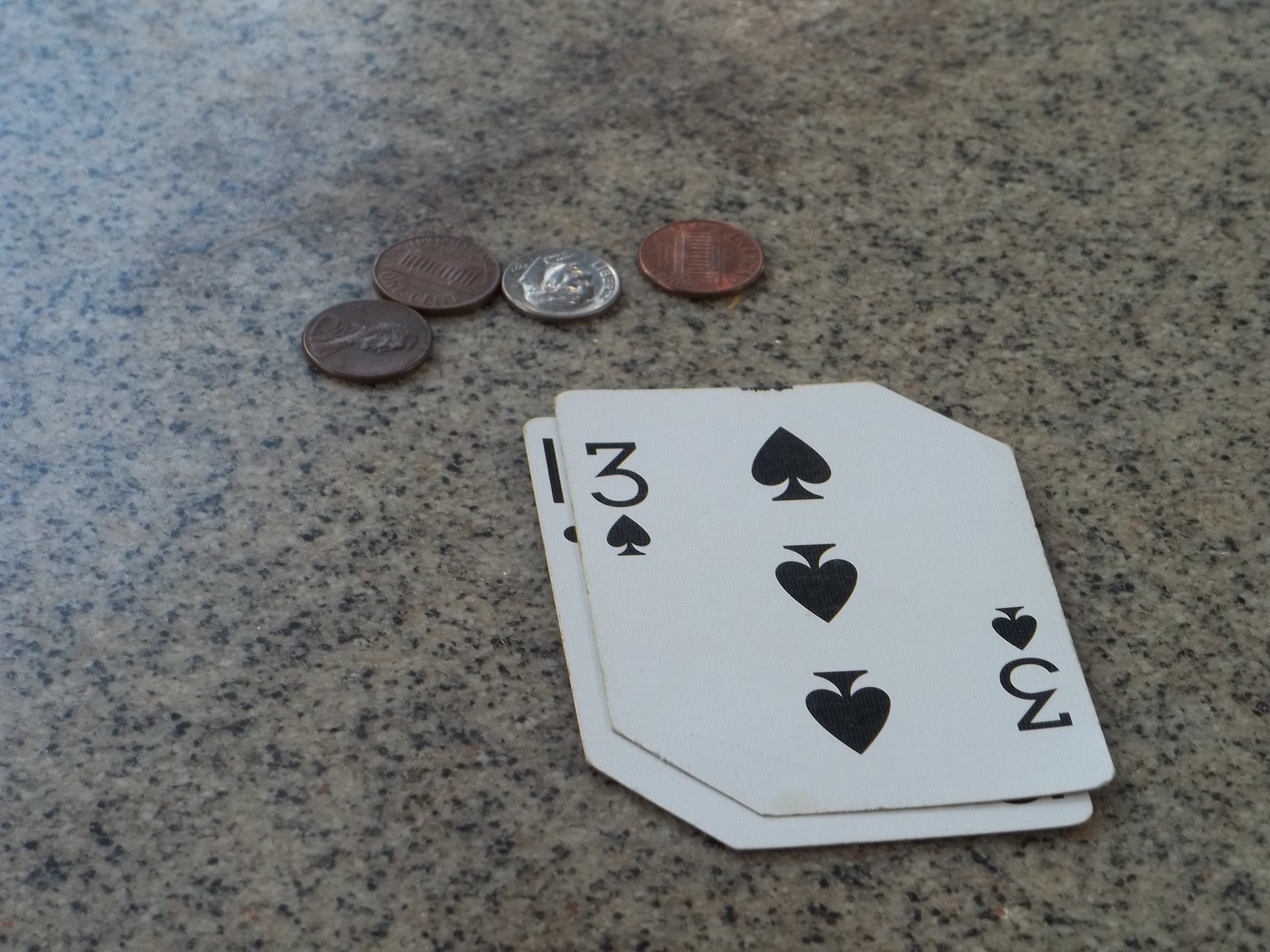In this detailed color photograph, a taupe table surface with brown and black speckles serves as the backdrop. At the forefront of the image are two playing cards stacked atop each other. The top card is the three of spades, clearly marked with black spade symbols on a white face. The bottom card displays only the number one, potentially also a spade, though its exact suit remains obscured. These cards feature a unique shape, characterized by rounded rectangles on two sides and clipped edges on the other two. Positioned just above the cards are four coins: three pennies and one dime. Two of the pennies are flipped tails-up, one is heads-up, and the dime is also heads-up. These coins rest slightly further back in the composition, creating a subtle depth against the speckled table surface.